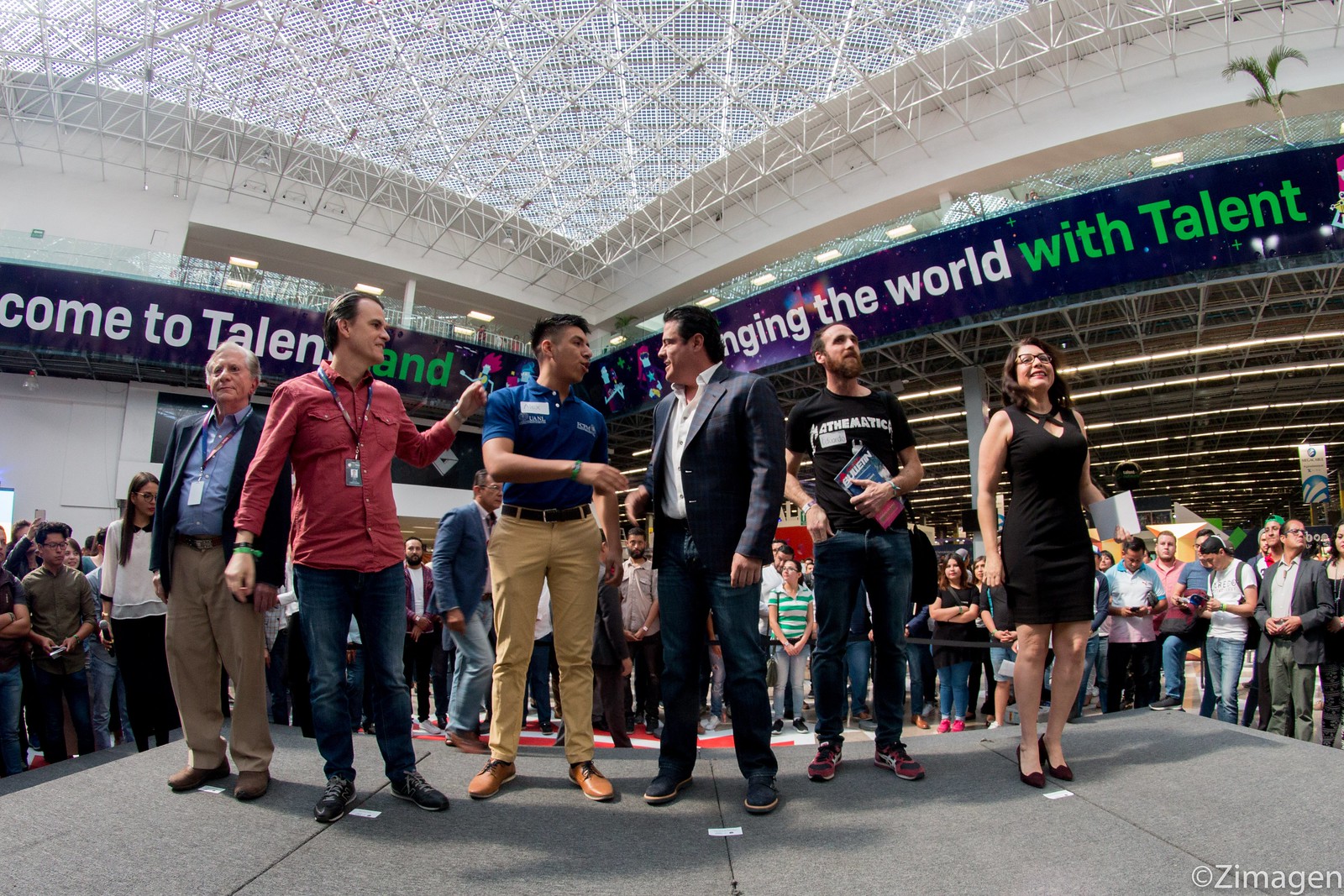This color photograph captures a dynamic scene at an indoor event, featuring six adults—five men and one woman—standing on a raised platform. The backdrop consists of a large, vaulted white-tile ceiling adorned with rows of lights, suggesting a vast indoor stadium. A crowd, dressed in jeans and business casual attire, fills the space behind and around the platform, adding to the event's bustling atmosphere.

A prominent banner reads, "Welcome to Talon" with the partial slogan "changing the world with talent." The people on the stage are primarily middle-aged, with one younger man. They engage in congratulatory gestures—shaking hands, touching shoulders, and conversing. Attendees on and around the platform face different directions, indicating a focus on various interactions rather than the camera.

The scene features a palette of colors, including green, dark blue, black, gray, white, light blue, coral, tan, beige, brown, and red. Additional details include name tags on the individuals on stage, various lighting fixtures, some bookers and plants in the background, and structural elements like poles and pillars. This detailed and vibrant photograph conveys a lively and well-attended event focused on talent and achievement.